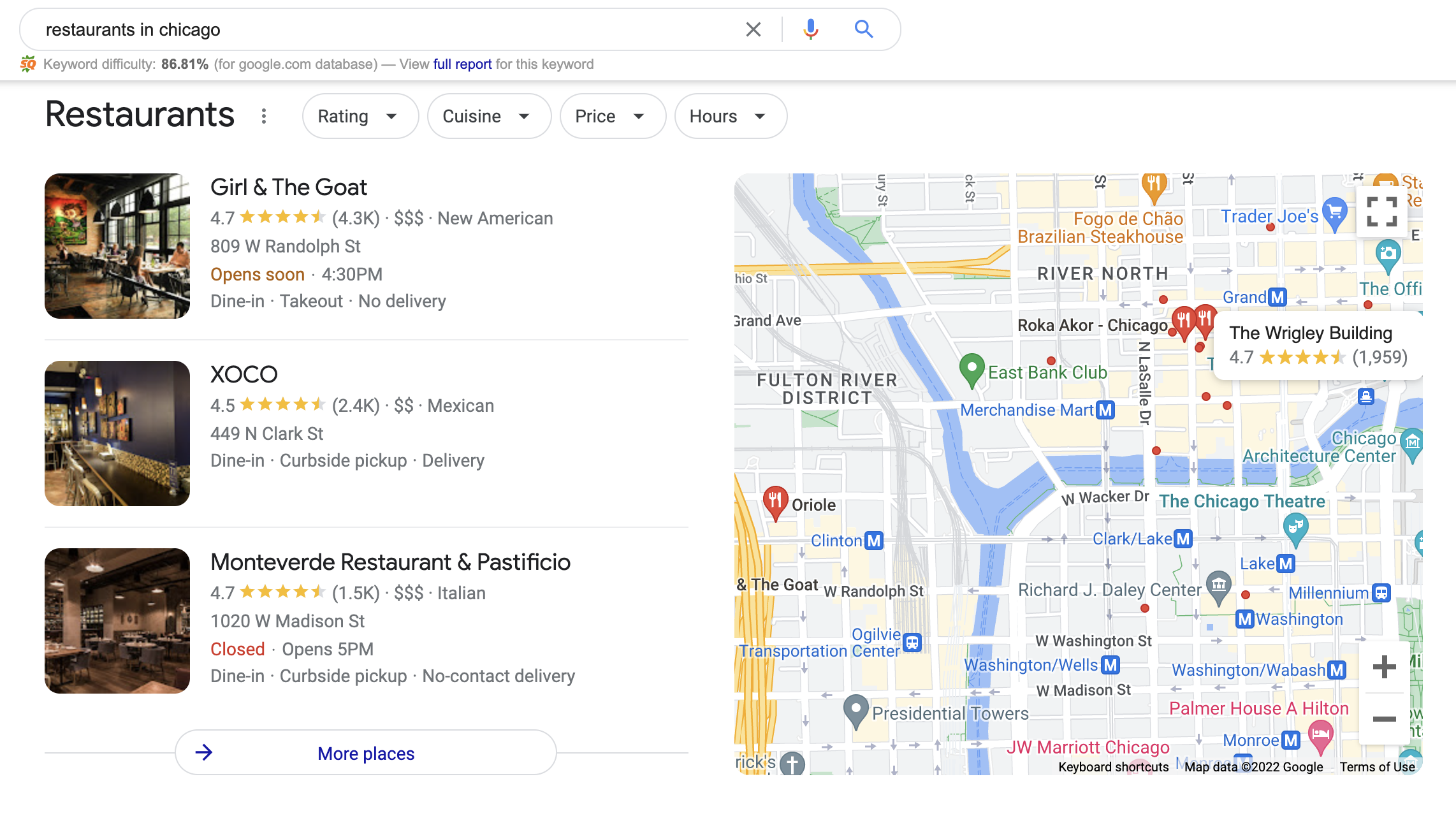The image showcases a webpage featuring a search bar at the top with the query "restaurants in Chicago." The keyword difficulty for this search is 86.81% according to the Google.com database, with an option to view the full report for this keyword.

Below the search bar, the page is organized into drop-down boxes labeled "Rating," "Cuisine," "Price," and "Hours," allowing users to refine their search parameters. On the far left of the page is a list of restaurant profiles, each accompanied by an image and detailed information.

The first listing is for "Girl and the Goat," which has a rating of 4.7 stars, based on 4.3K reviews. It is categorized with three dollar signs, indicating a higher price range, and serves New American cuisine. The address is 809 W West Randolph Street. It opens soon at 4:30 p.m. and offers dine-in and takeout options, but no delivery.

Next is "Zoco," which is prominently displayed in capital letters. It has a rating of 4.5 stars from 2.4K reviews. Marked by two dollar signs, this restaurant provides Mexican cuisine and is located at 449 North Clark Street. Zoco offers dine-in, curbside pickup, and delivery services.

The third featured restaurant is "Monteverdi Restaurant and Pestificio," boasting a 4.7-star rating based on 1.5K reviews. With three dollar signs, it falls into the higher price range and serves Italian cuisine. Located at 1020 West Madison Street, it is currently closed but will open at 5:00 p.m. Monteverdi offers dine-in, curbside pickup, and no-contact delivery services.

At the bottom of the listings, there is an option labeled "More Places" for further browsing.

On the far right side of the page, a map displays the area with symbols indicating various restaurants and other points of interest.